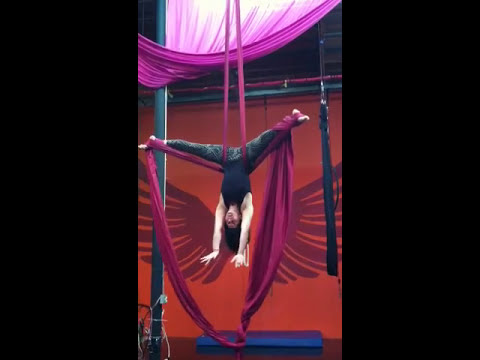The image captures a dramatic scene of a performer engaged in an aerial act, suspended upside down by magenta cloth ropes with legs splayed apart. She is wearing a black tank top and dark gray leggings, her black hair falling towards the safety mat below. The background features an orange wall adorned with two large, darker purple wings painted behind her, giving an ethereal effect. Gray support poles are visible, with one notably positioned near her right foot. Above her, violet and white drapery adds to the intricate setup. The performer appears to be in the middle of a circus or acro yoga performance, gracefully managing the magenta rope entwined around her ankles. The stage is framed by black bars on either side, and a blue safety mat rests at the bottom, emphasizing the athleticism and safety considerations of the performance.